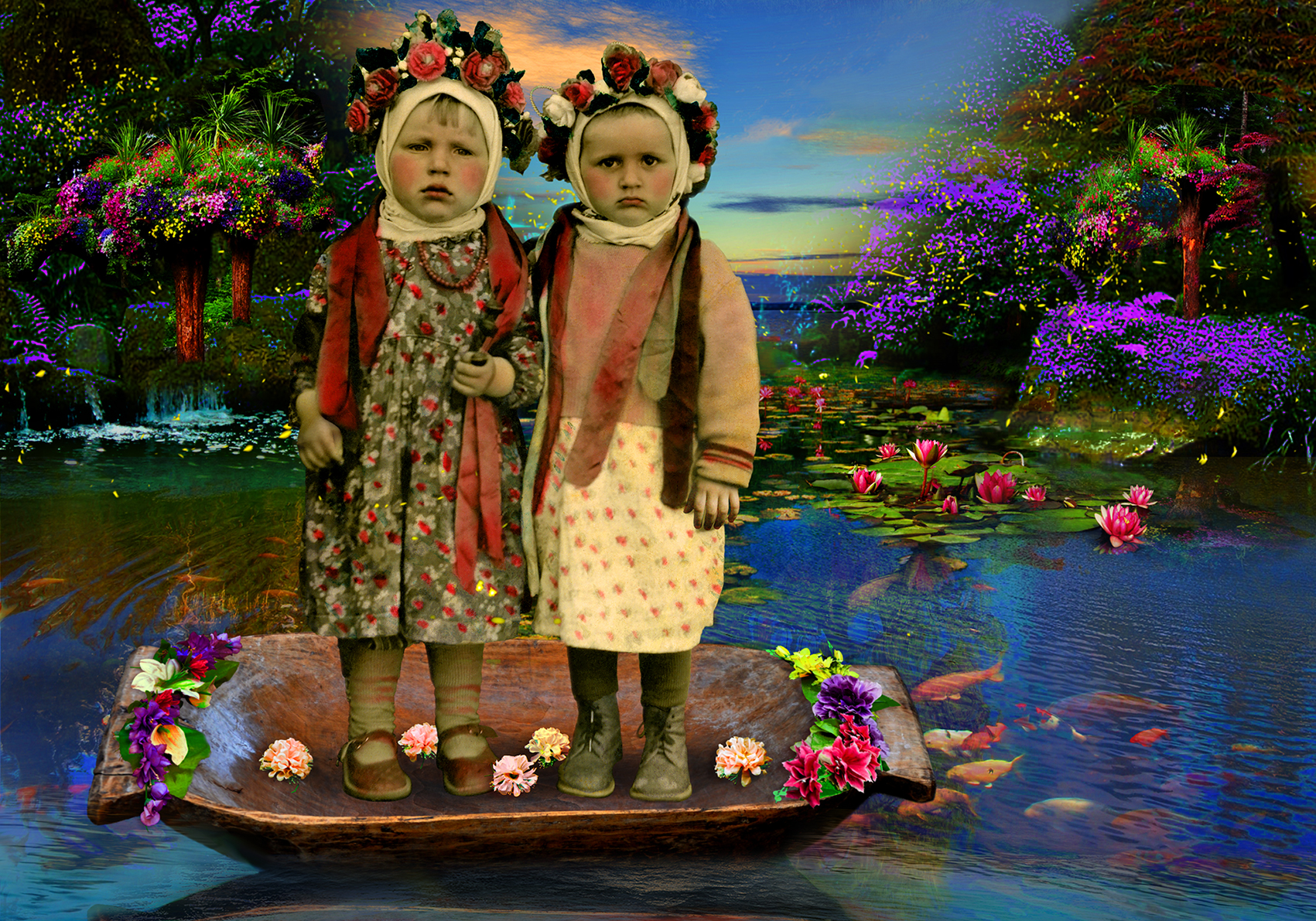In this surreal, dreamlike painting, two young children stand stoically in the center of a tiny, wooden canoe adorned with vibrant flowers. The canoe, seemingly hewn straight from a tree, is surrounded by a clear, bright blue pond filled with swimming koi fish beneath the surface. The children, both appearing to be around five years old, have distinct, unhappy expressions with scowls on their faces. Their faces are an unusual gray tone with a hint of pink on their cheeks, contributing to the fantastical atmosphere.

Both children wear white towels wrapped around their heads like turbans. The child on the left is dressed in a green floral dress with a red scarf draped over their shoulders, while the child on the right dons a yellow floral dress, green socks, green boots, and a vest that transitions from pink to a brown-gray hue. Flowers also adorn their heads, adding to the whimsical scene. 

The background bursts with color: purple and pink flowers, lush green bushes, and vibrant trees frame the scene. The sky above is a bright blue with a few sunlit clouds, and there are patches of land on either side filled with flowers and greenery. Floating on the water behind the children are green lily pads, each supporting a striking red flower. The landscape beyond the immediate scene seems infinite, merging water and sky in a dreamy, fairy-tale garden setting.